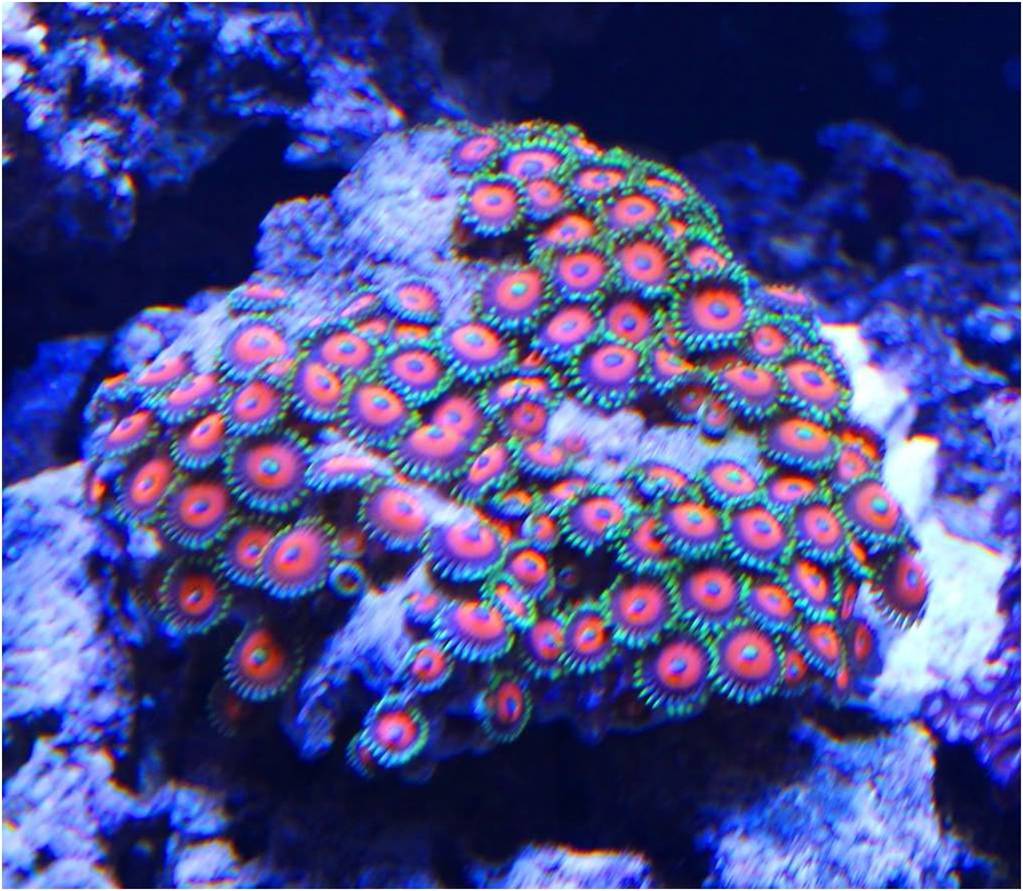In this underwater photograph, various vividly colored corals are prominently displayed in the foreground. The corals showcase a mesmerizing spectrum of colors: primarily greens, purples, reds, and blues. Each coral has a distinct pattern, often featuring a green outline with a red circle and a blue dot at its center. Some corals display additional intricate details, with a mix of purples and reds interspersed within the green borders. These corals, gathered densely together, rest on what appears to be a rocky coral reef formation. The clear, blue-hued water in the background accentuates the peaceful and calming atmosphere of this underwater scene, devoid of any marine life other than the corals themselves. The natural design and vivid colors of the corals create a serene and enchanting visual experience.